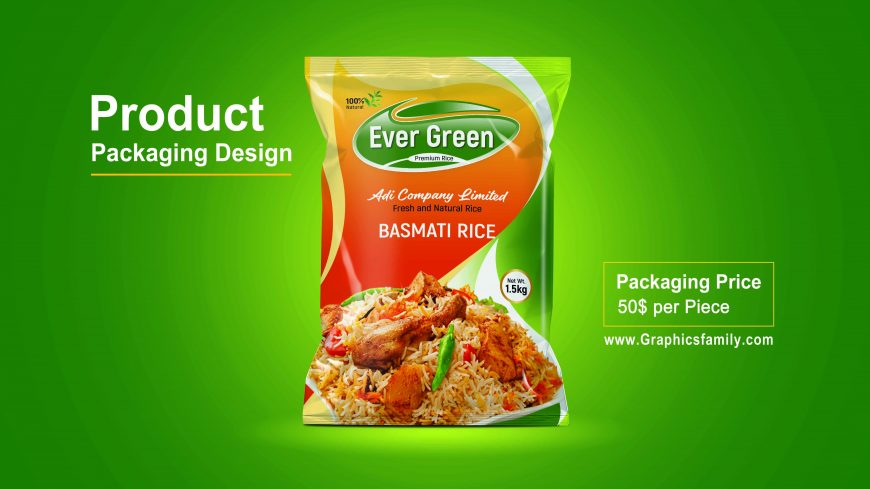The image showcases a vividly designed product packaging for Evergreen Basmati Rice from Addy Company Limited. The central feature is a detailed depiction of the rice bag, which stands out against a predominantly bright green background interspersed with darker green accents. The top section of the bag features a mix of orange, red, and green colors. Prominent on the bag are the brand name "Evergreen" in bold white text against a green background, the company name "Addi Company Limited," and the product details including "Fresh and Natural Rice" and "Basmati Rice." The net weight of 1.5 kg is displayed on the right side. Also prominently featured is a mouth-watering image of a dish containing yellow rice, brownish meat, and green beans, neatly presented on a white dish. On the left side of the picture, the text "Product Packaging Design" appears in white with a yellow underline. To the right, a yellow rectangle highlights the text "Packaging Price $50 per piece" with the website "www.graphicsfamily.com" below, indicating that this may be an advertisement for a packaging design service.